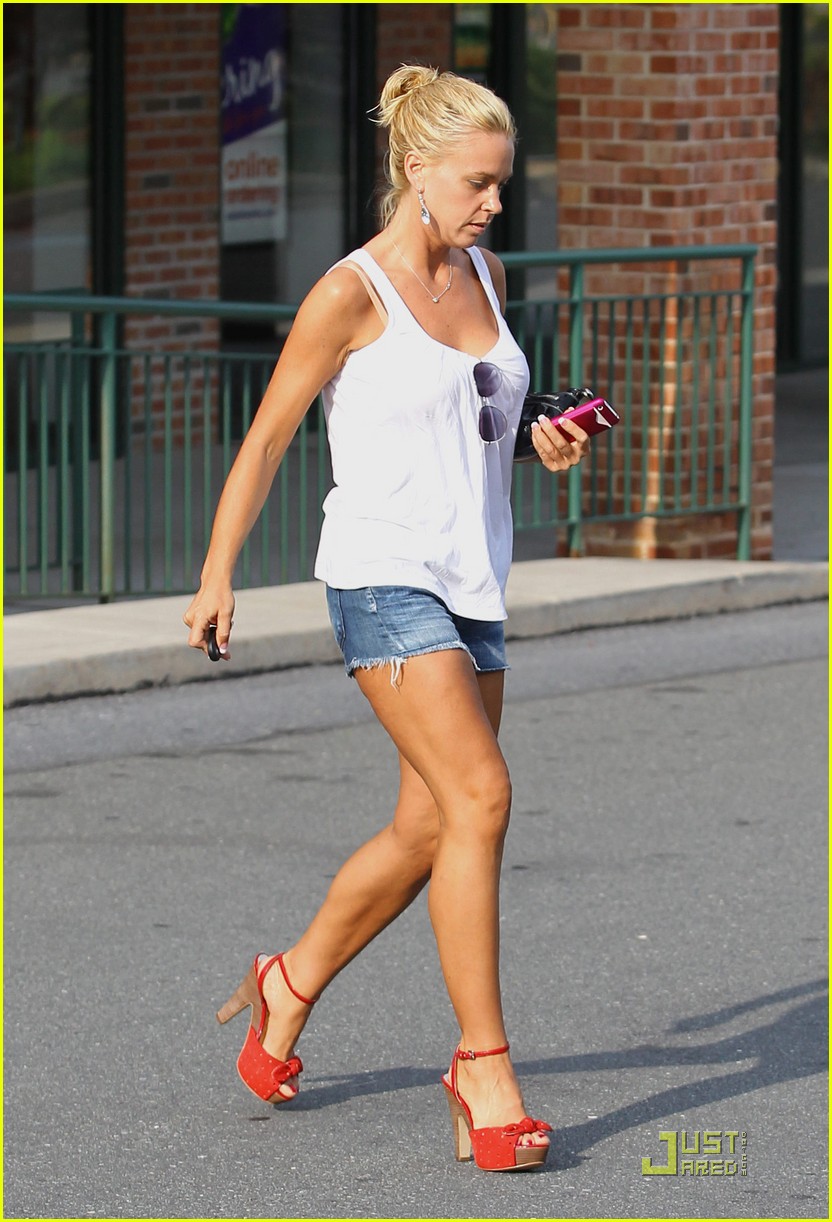A blonde, tan woman in her 40s is crossing a gray roadway, situated in the middle of the image and walking towards the right. Her hair is tied up in a ponytail, and she looks down at the ground. She wears silver dangle earrings, a silver necklace, and a white tank top that shows a visible skin-tone bra strap. Aviator sunglasses are tucked into her tank top. She has on very short denim shorts or a skirt, showcasing her long legs, and red high-heel sandals. She holds a purple phone and maybe headphones in one hand, and her car keys in the other. The background features a green railing, windows, and brick pillars of a store, indicating a parking lot setting. The image includes a watermark at the bottom that reads "JustJared.com" in green.